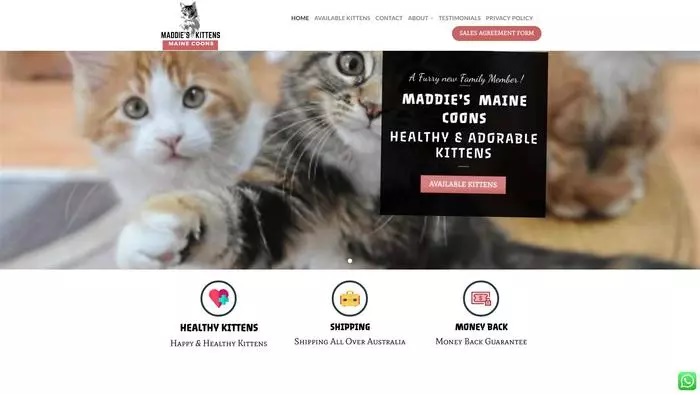The webpage is dedicated to kittens and prominently features the title "Maddie's Kittens" at the top. The navigation menu includes options such as Home, Available Kittens, Contact, About, Testimonials, Privacy Policy, and a Sales Agreement Form. All menu items are in black text, except for the Sales Agreement Form, which stands out with white text on a red background.

Below the navigation bar, a large image showcasing three cats is displayed. The first cat is orange and white, the second is a dark-striped tabby, and the third cat’s white belly and orange-and-white paws are partially visible. Overlaying this image, white text reads: "A furry new family member," alongside "Maddie's Maine Coons: Healthy and Adorable Kittens" and "Available Kittens." The words "Available Kittens" are set against a pink background while the rest of the text is on a black box.

Further down, the page promotes three key features: Healthy Kittens, Shipping, and Money Back. Each feature is enclosed in black-bordered circles. Under Healthy Kittens, the text "Happy and healthy kittens" is written in black, accompanied by an icon of a pink and red heart with a blue plus sign. The Shipping section contains an icon of a yellow suitcase and mentions "Shipping all over Australia." The Money Back section guarantees "Money back" with an icon displaying pink dollar signs and a pink cash bag.

Near the bottom of the page, there is a green phone icon enclosed in a circle, likely indicating a method for contacting them.